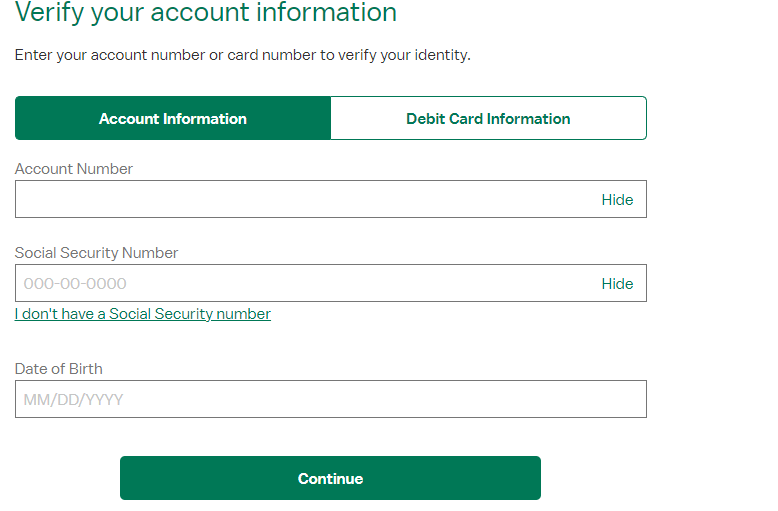The image depicts an account verification area. At the top left corner, in green font, it says "Verify Your Account Information." Below this, it instructs users to "Enter your account number or card number to verify your identity." 

On the left side, there is a dark green rectangle button labeled "Account Information." To the right, there is a white button labeled "Debit Card Information," with the label in green font.

Further down, there is a section labeled "Account Number" in faded gray font. Adjacent to it is a long rectangular input box with the word "Hide" on the right side. Below this section, "Social Security Number" is mentioned with another input box filled with example zeros, and "Hide" again on the right-hand side. A note reading "I don't have a Social Security Number" is underlined and in green font.

The next section is labeled "Date of Birth," followed by a long rectangle box with the placeholder text "mm/dd/yyyy" in faded font. 

At the bottom of the area, there is a space of white, followed by a long rectangular green button labeled "Continue" prominently in the center.